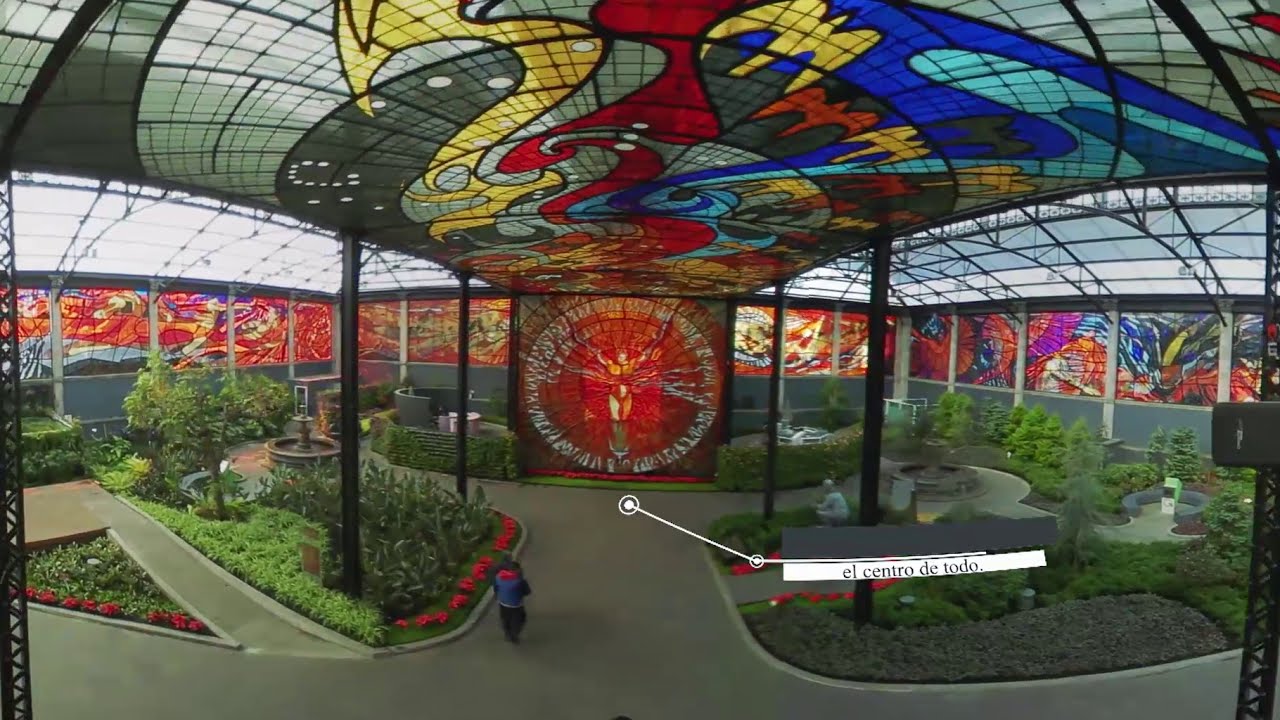This detailed image captures an indoor park abundant with greenery, featuring a myriad of plants, flowers, trees, and small bushes. There are multiple pathways, diverging left and right into three paths each, all intricately lined with various colorful shrubs and neat, attractive plant beds. Two people populate this space: one man wearing a blue top and black bottoms walks down a central path towards the focal point of the park, while another person sits on a bench to the center-right.

At the heart of the image, a large, striking stained glass window, prominently centered, showcases a figure with arms raised, crafted with hues of red, orange, and clear glass. This window is set amidst hedges and other greenery, and a pathway leads directly to it. Above, the ceiling and upper walls are adorned with additional stained glass mosaics in vibrant reds, blues, yellows, purples, and blacks, allowing natural light to filter through, casting colorful patterns across the space.

A noteworthy detail is a white banner featuring black text, reading "El Centro de Todo," located on the center-right of the image. This banner is connected to a thin white line and dot formation, both above and below. The overall ambiance is further enriched by small water fountains strategically placed on both sides, adding to the serene, indoor garden atmosphere of this beautiful, daylit space.